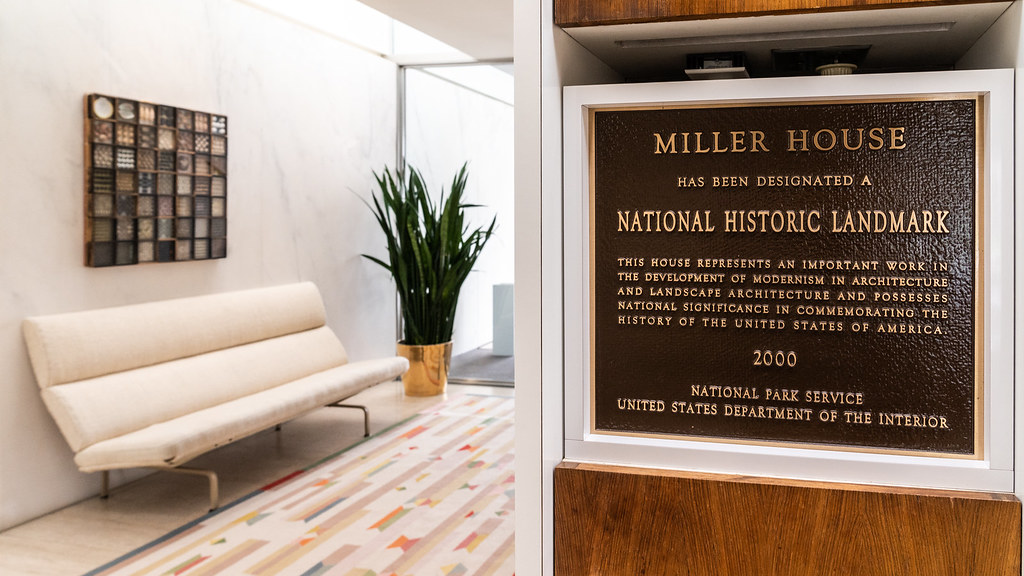The photograph showcases a modern interior split into two distinct sections. On the right side, a metal plaque with a white border is embedded in a white wall with wooden accents. The plaque, set within a wardrobe-like fixture, announces that Miller House has been designated a National Historic Landmark by the National Park Service in 2000 for its significance in the development of modernism in architecture and landscape architecture. To the left, an elegantly styled waiting area features a white leather lounge sofa placed against a wall adorned with a decorative piece of art. A large, shiny golden pot holding a spiky green plant stands beside the sofa. The floor boasts a colorful Navajo-patterned rug over a likely vinyl wood surface. A glass window is positioned behind the plant, allowing a glimpse into an adjacent room, enhancing the sense of openness and light in the space.